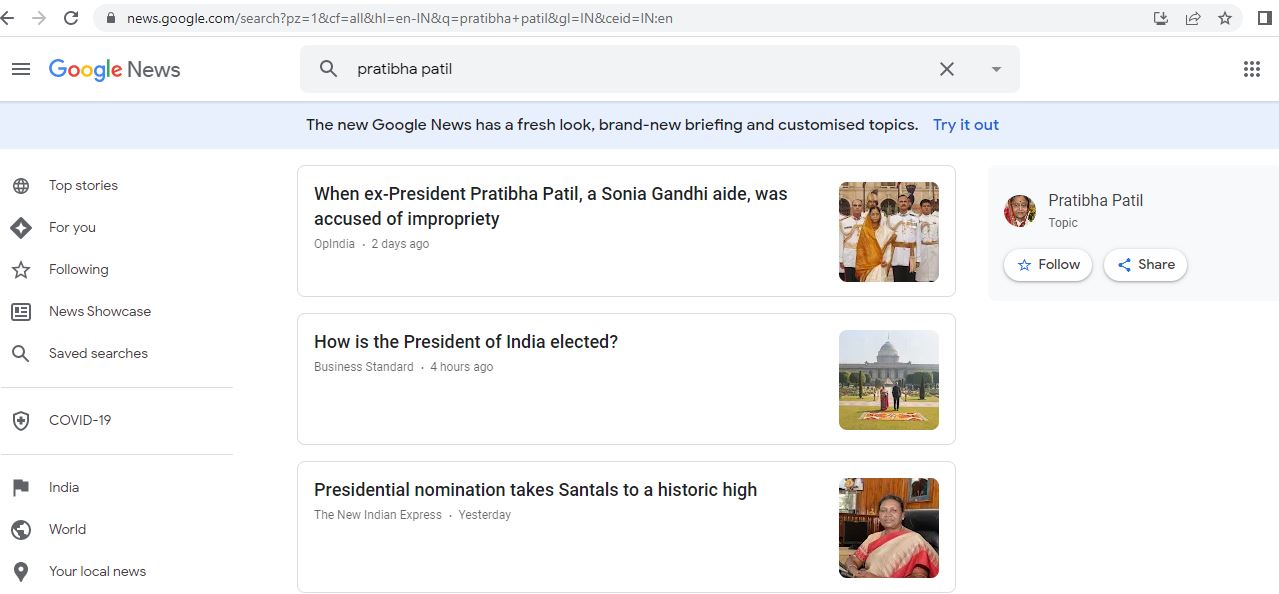**Google News Interface Overview: Pratibha Patil Story Highlight**

The image captures a detailed view of the new Google News website interface. At the top, navigation arrows and a refresh bar are visible, followed by the URL "news.google.com". The search query contains parameters specific to a news search about "Patel," with filters for localized Indian content and English language preferences.

A prominent blue notification banner highlights the new features: "The new Google News has a fresh look, brand-new briefing, and customized topics. Try it out."

Below, sections are organized with categories like:
- Top Stories for You
- Following
- News Showcase 
- COVID-19 updates
- India, World

A segment on local news is also provided.

The main news story featured is about ex-president Pratibha Patil and mentions Sonia Gandhi, referring to an incident of "impropriety" in India from two days prior. A photograph shows several individuals standing around. The news snippet suggests options to follow or share the topic "Pratibha Patil."

Additional snippets include:
- An article discussing "How has the president been elected" from "Business Study" published four hours ago with imagery of a building and lawn.
- A headline about "President Trump nomination" noting a "strike high" from "The New Indian Express" published the day before.

The interface emphasizes a customized experience with up-to-date briefings and a sleek design.